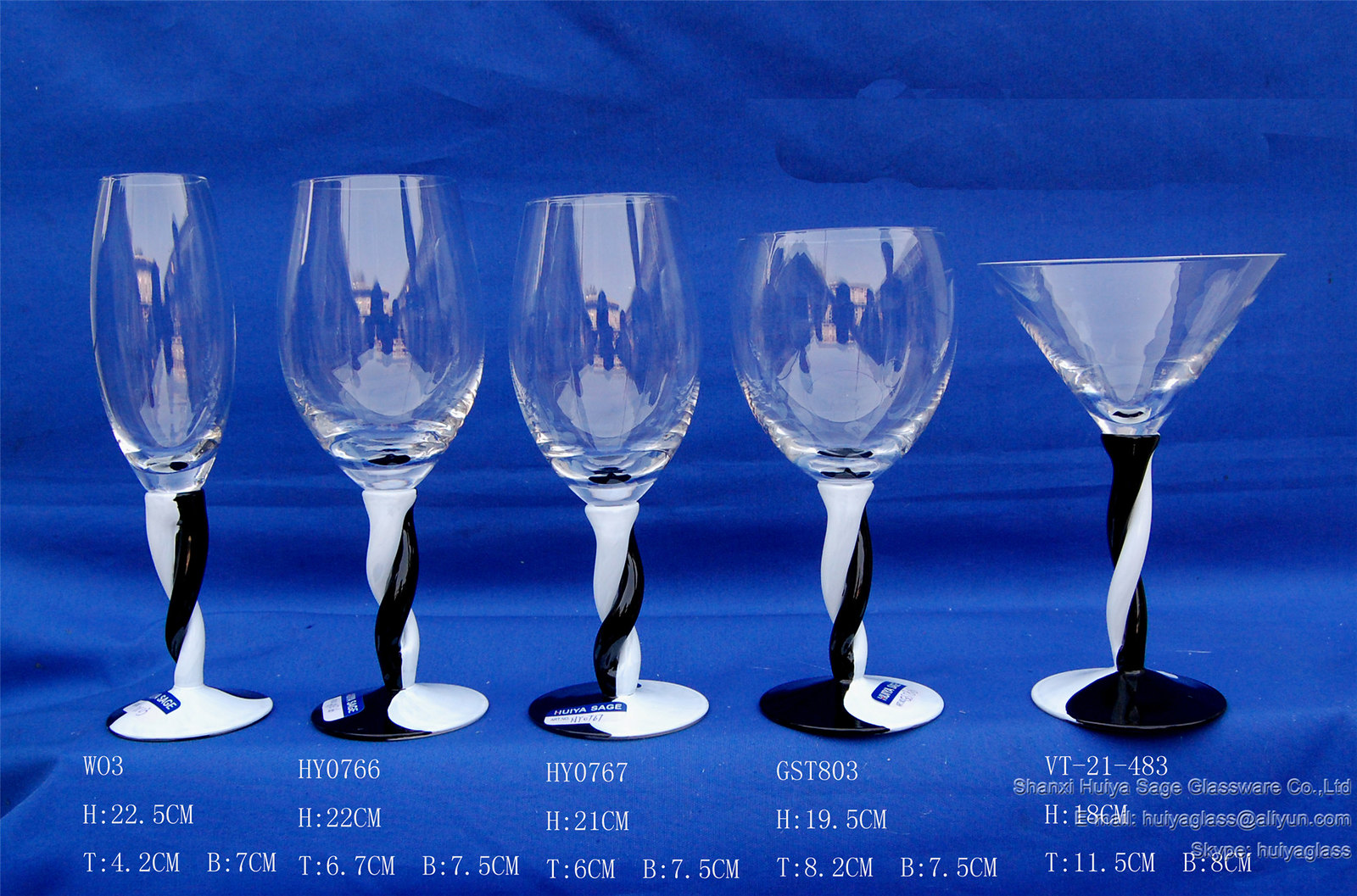The image features a catalog or advertisement page from Shanzhi Hulie Sage Glassware Company Limited, set against a rich royal blue background. Displayed are five distinct glasses arranged from tallest to shortest. The glasses, used for wine, champagne, and martinis, showcase clear glass receptacles on top of twisted black and white stems that resemble intertwined ribbons, giving a yin-yang appearance. The bases of these stems follow the same two-tone pattern. Below each glass, white text specifies their catalog numbers and dimensions, such as "W03H 22.5CM T 4.2CM B 7CM." The background cloth is also blue, adding depth to the display. Blue and white informational stickers are affixed to the bases of the glasses, indicating details about Sage Glassware Co. LTD, visible at the bottom right of the image.